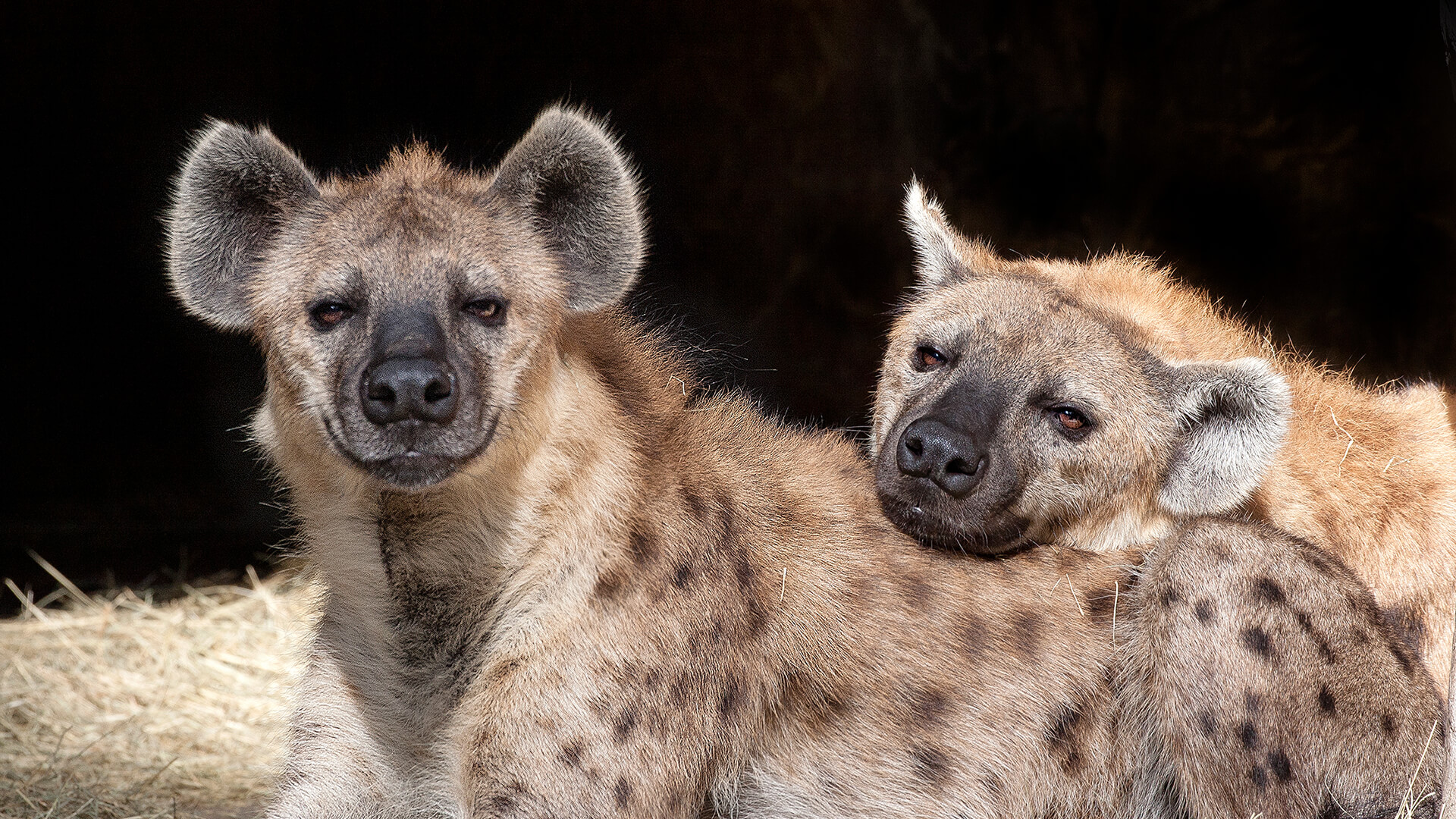In the photograph, two hyenas are lounging in the sun against a stark black background. The hyena in the foreground is positioned in the center of the image, displaying a relaxed demeanor with light brown fur speckled with darker spots. Its ears and mouth area are a darker black, and it has dark brown ears that stick out prominently. The creature's face, framed by folds that suggest a smile, is marked by dark eyes and a nose that contrasts with its lighter fur. This hyena has a slight mohawk and is looking directly at the camera with a seemingly relaxed expression.

Behind this hyena, slightly to the left, lies the second hyena, which rests its head on the back of the first. This second hyena appears grayer and somewhat lighter, possibly due to the sunlight casting a tan hue on its fur. Its features include similar big, round ears with grayish fuzz and it looks into the distance, contributing to a serene scene. The background features a stack of hay on the bottom left, adding a touch of natural habitat to the otherwise obscured backdrop. Overall, the image captures a moment of tranquility between the two hyenas, highlighted by their distinctive markings and relaxed postures.